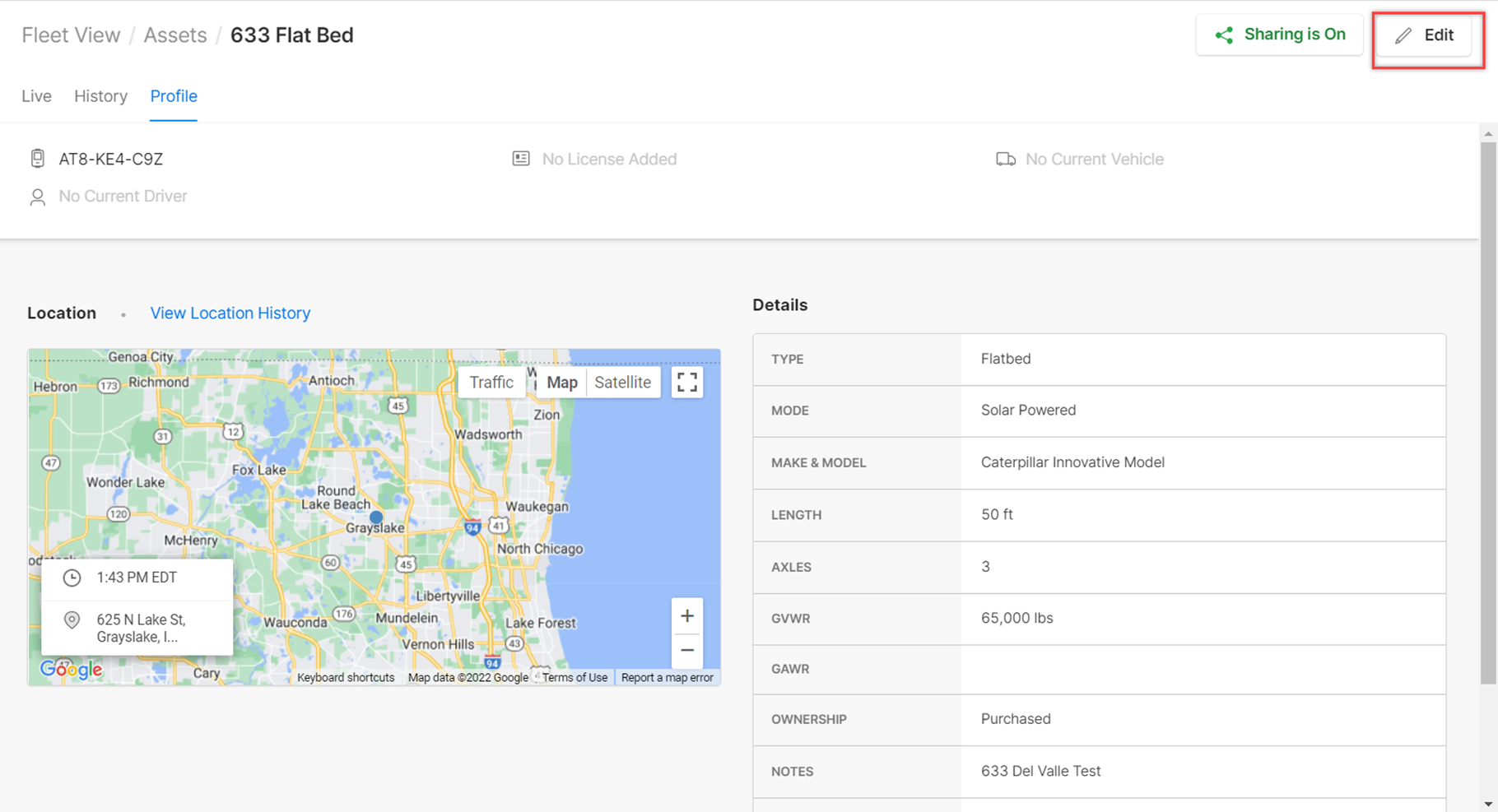**Detailed Caption:**

The screenshot depicts a user interface titled "Fleet View" with a specific asset labeled as "633 Flatbed." The information at the top right indicates that "Sharing is on," highlighted within a white box using green text. Below this, there is a red rectangle enclosing the "Edit" option accompanied by a pencil icon, alongside menu options like "Live," "History," and "Profile."

Further down, a map interface details the geographical area encompassing North Chicago, Lake Forest, Vernon Hills, and Forest Lake. 

The asset information section specifies attributes such as:
- Mode
- Type
- Model
- Current vehicle status (none)
- Licenses added (none)
- Current driver (none)

Additionally, a possible identifier resembling a license plate reads "AT8/AE4/CZ."

The map features a pinpoint indicator showing the vehicle's last known location and offers viewing options including traffic and satellite modes. Users can also zoom in or out for a closer or broader map perspective.